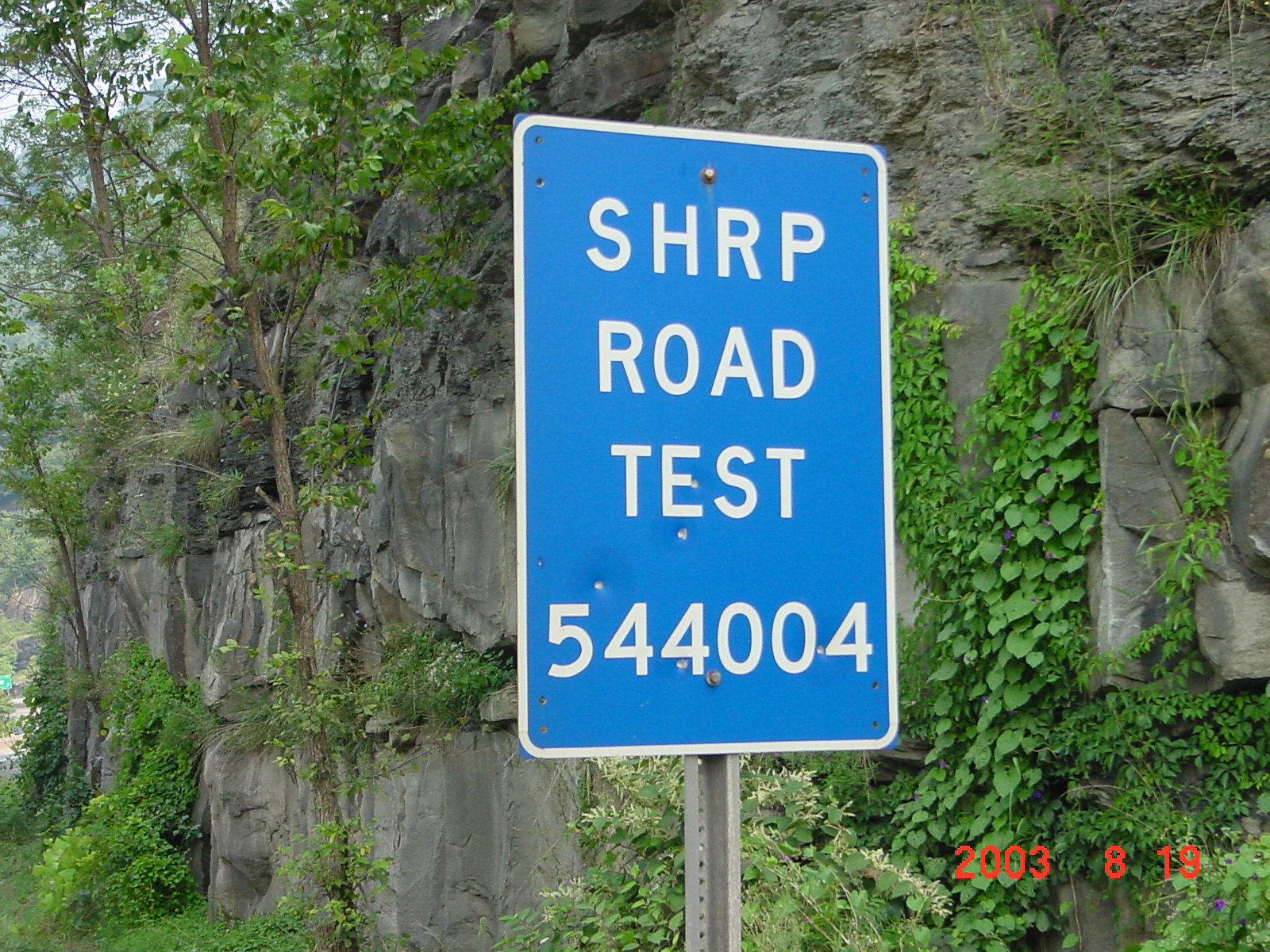The photograph vividly captures a road sign mounted on a silver metal pole. The rectangular sign is a dark blue-green color with white writing that reads "SHRP Road Test 544004," encased by a whitish outline. In the bottom right corner of the image, a red timestamp reads "2003-8-19." The sign stands in front of a rocky cliff that extends upward beyond the frame, characterized by a smooth lower section that becomes rockier with more pronounced edges toward the top. The cliff face is adorned with greenery, including overgrown grass at the base, vines climbing upward, and a variety of long thin trees with green leaves. There are hints of purple flowers among the foliage, and the upper left corner of the image reveals a small patch of blue sky visible through the tree canopy. The overall scene is set against the backdrop of a gray rock wall with some darker shades, providing a textured contrast to the lush vegetation.